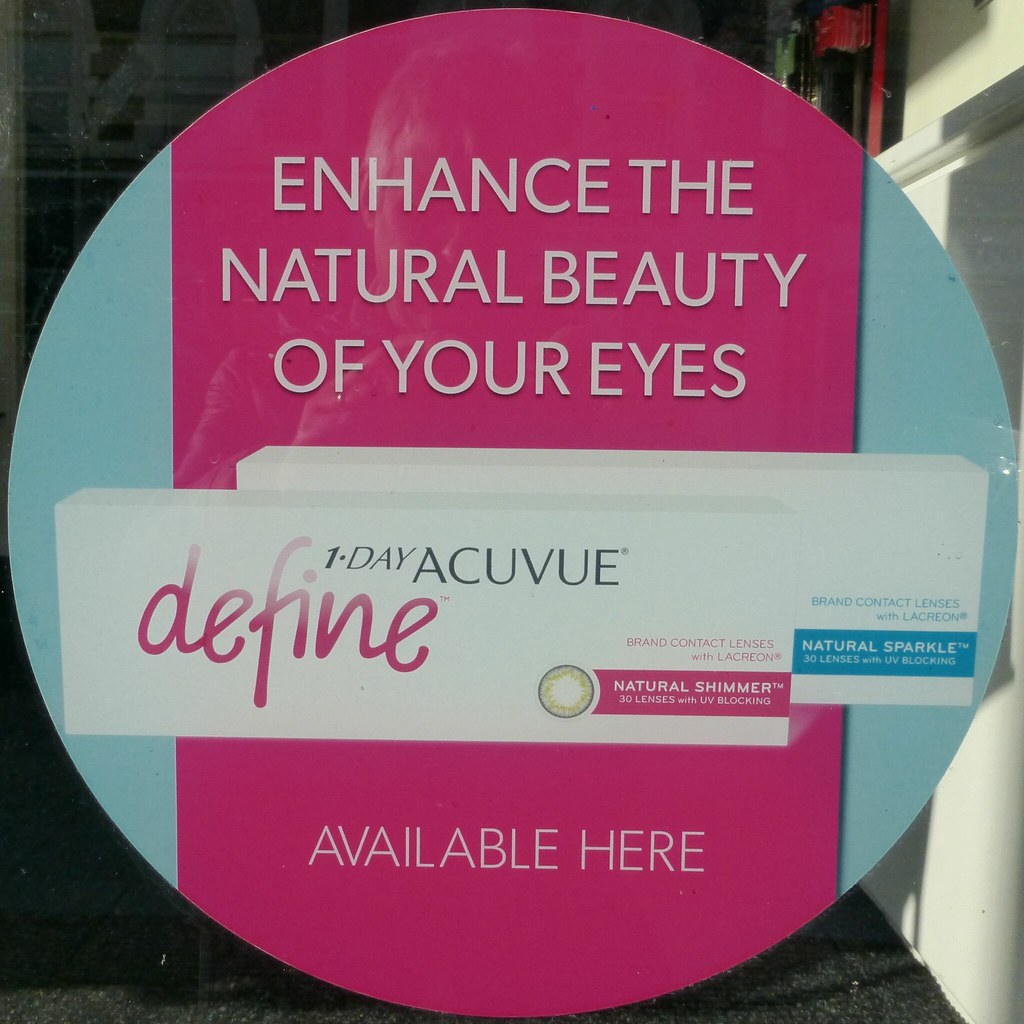The image is a detailed advertisement for Acuvue Define 1 Day Brand Contact Lenses. The ad is dominated by a large central circle with a bright pink top and light teal edges. Over the pink background, white text reads, "Enhance the natural beauty of your eyes." Below, the text "Available here" is displayed in blue with white letters. In the middle of the circle, an image of a box for the contact lenses is prominently featured. The box features black text that says "1 Day Acuvue" and cursive black text that reads "Define." To the right in pink letters, it states, "Brand Contact Lenses with Lacreon." Beneath it, in a pink rectangle with white text, it says, "Natural Shimmer, 30 lenses with UV Blocking." Adjacent to this main box, another similar box is visible, with the main difference being a teal rectangle stating "Natural Sparkle, 30 lenses with UV Blocking." The room's background is minimal, showing only a gray floor and white wall, emphasizing the product's vivid and colorful presentation.